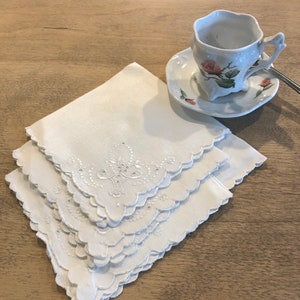This detailed photograph features a vintage-style white porcelain teacup and matching saucer, both adorned with red roses and green leafy vines. The teacup, which has a somewhat irregular, rounded shape, is positioned in the top right of the image. A small teaspoon rests against the side of the teacup, which appears empty. The teacup and saucer set is elegantly placed on a medium-brown wooden table. In the center-left of the image, there is a stack of four meticulously folded white napkins, neatly arranged in a diamond pattern. Each napkin features a white fleur-de-lis design with glossy thread accents. The napkins have two straight edges and two rounded edges, giving them a decorative look. This simple yet refined setup is presented against the backdrop of the wooden tabletop, making the vintage teacup and the carefully folded napkins the focal points of the photograph.